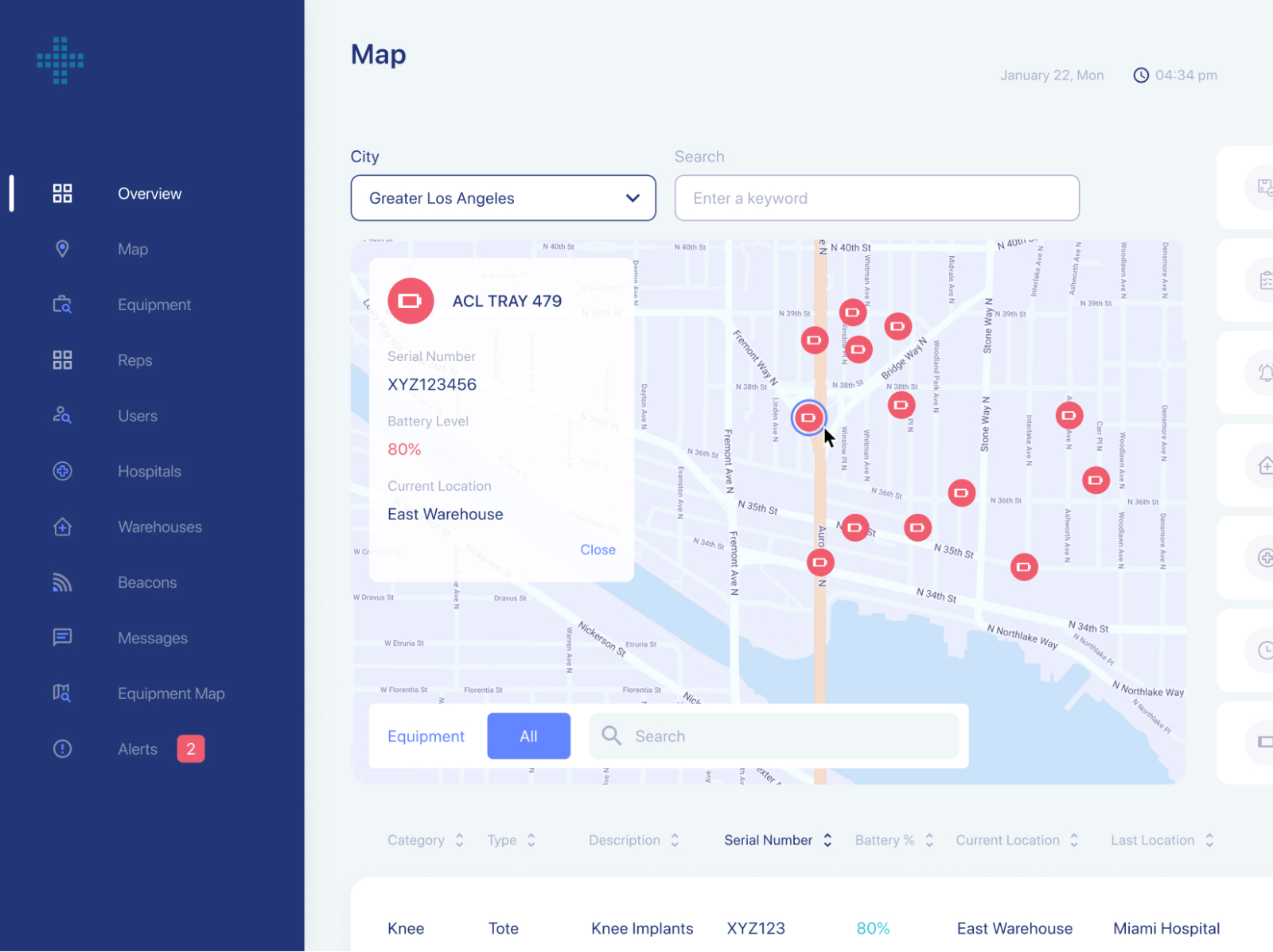Screenshot of a dashboard interface displaying a detailed map of Greater Los Angeles. The page is divided into multiple sections. On the darker royal blue left-hand side column, there is a vertical menu listing ten options: Overview, Map, Equipment, Reps, Users, Hospitals, Warehouses, Beacons, Messages, Equipment Map, and Alerts. 

To the right, occupying the majority of the screen, is a map section. In the top left corner of this section, it is labeled "Map." The map itself has a light grey background with streets and avenues depicted in white, labeled in black text, and a light lilac backdrop. A blue-colored river can be seen running through part of the map, adding a distinct feature to the area. Scattered across the map are approximately a dozen small, round red markers indicating specific locations of interest.

One red marker is highlighted in blue and features an arrow pointing to it. A pop-up window adjacent to this highlighted marker provides detailed information, indicating it is "ACL Tray 479" along with its serial number, battery level, and current location. This highlights the interactive and detailed nature of the dashboard, designed for monitoring and managing equipment and locations efficiently.